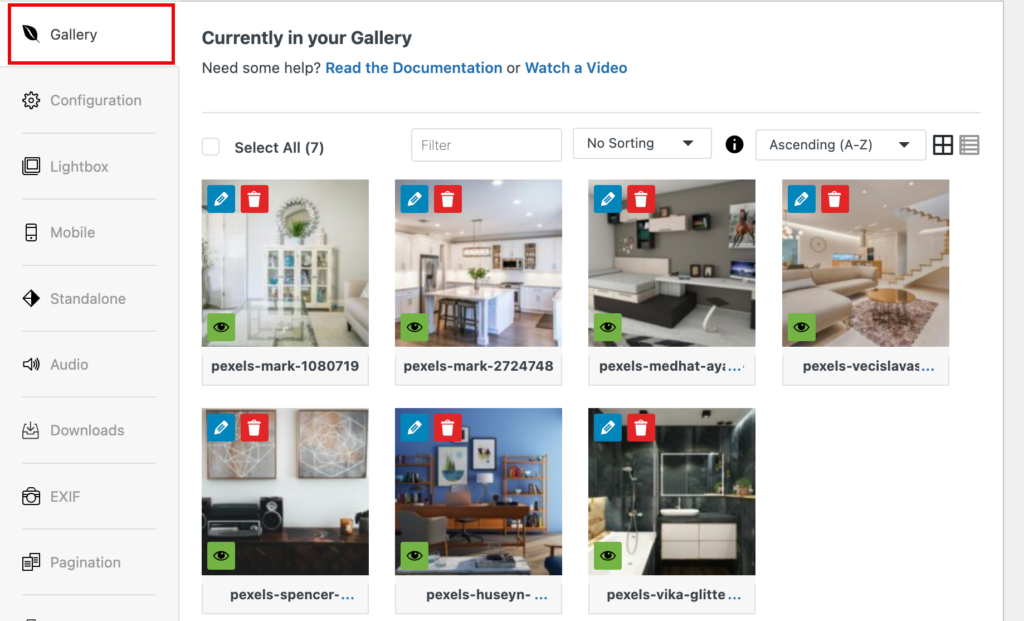Screenshot of user's gallery interface showing a collection of seven distinct interior design photos, each outlined in red. 

1. First image: A white living room cabinet with double doors.
2. Second image: A modern kitchen featuring built-in appliances and large counter spaces, with a microwave integrated into the wall and a central counter table.
3. Third image: A multifunctional bed that doubles as a desk, labeled with "Pexels Mark".
4. Fourth image: A cozy living room with brass-topped table, two loveseats, and double set of stairs.
5. Fifth image: An entertainment center with a stereo system, flanked by two paintings above.
6. Sixth image: A study desk adorned with multiple books and organized racks.
7. Seventh image: A luxurious black marble bathroom, equipped with a large mirror, sink with a stand, and an adjustable spray showerhead.

The gallery webpage appears to offer options for configuration, lightbox, mobile view, standalone features, audio downloads, EXIF data, and pagination.